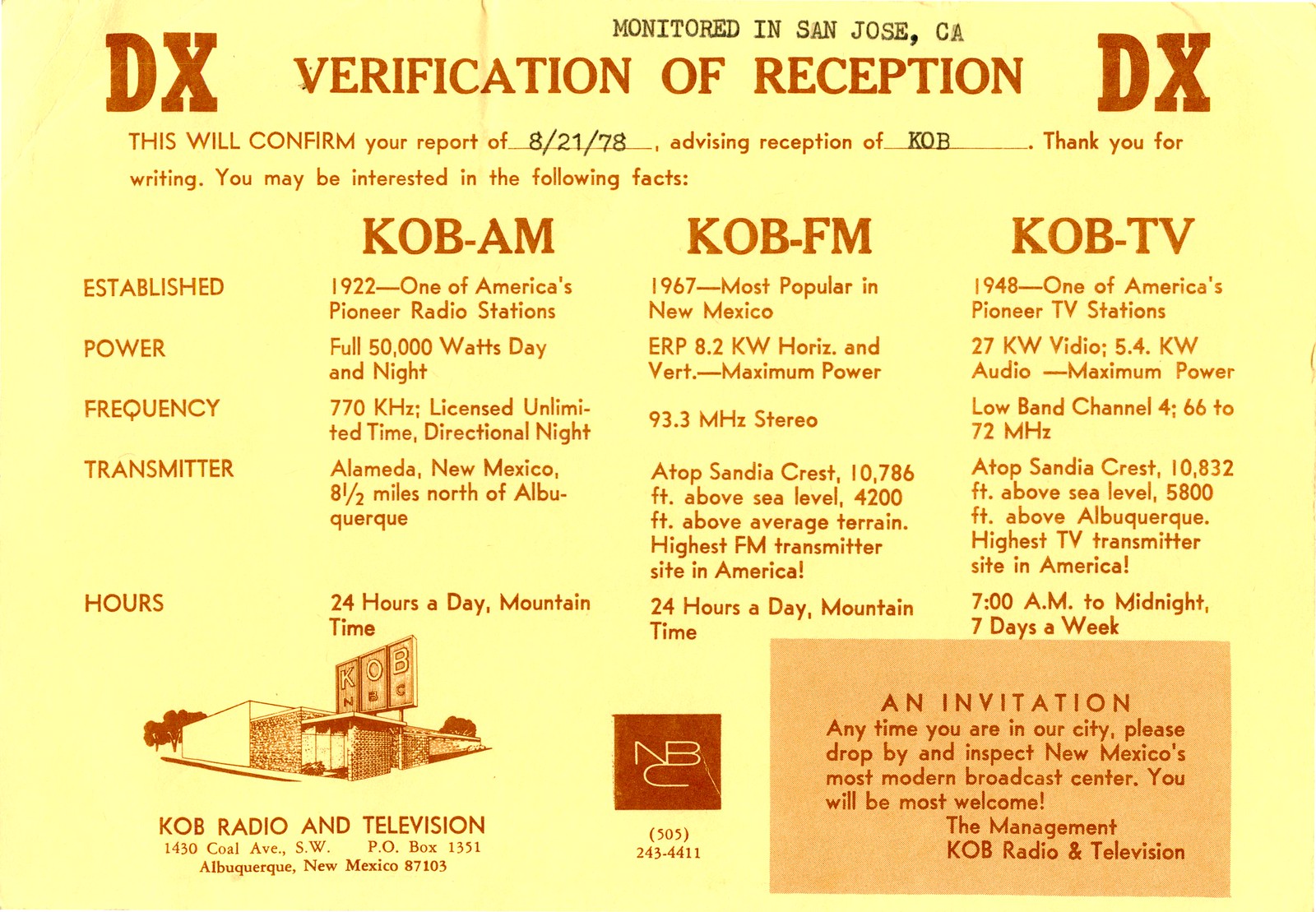The image appears to be a vintage-style receipt or verification form, set against a yellow background with brown text and logos. At the top, within a white background, it reads "Monitored in San Jose, California," followed by the heading "Verification of Reception" prominently displayed with the letters "DX" flanking either side. The form confirms a report from August 21, 1978, acknowledging the reception of the KOB broadcast. The text expresses gratitude for writing and offers various facts about KOB's broadcasting stations.

On the left, the document details KOB-AM: established in 1922, one of America's pioneer radio stations, broadcasting powerfully at 50,000 watts day and night on a frequency of 770 kilohertz. The transmitter is located in Alameda, New Mexico, about 8.5 miles north of Albuquerque, with operational hours spanning 24 hours a day, Mountain Time.

Next, it discusses KOB-FM, established in 1967, noted as the most popular FM station in New Mexico. It operates at 8.2 kilowatts ERP on a frequency of 93.3 megahertz in stereo, with the transmitter positioned atop Sandia Crest, the highest FM transmitter site in America at an elevation of 10,786 feet above sea level. This station also runs 24 hours a day, Mountain Time.

Additionally, the form includes information about KOB-TV, established in 1948 and described as one of America's pioneer TV stations. It broadcasts with 27 kilowatts video and 5.4 kilowatts audio power on low-band channel 4 (66 to 72 megahertz). Its transmitter is also located atop Sandia Crest at 10,832 feet above sea level. KOB-TV operates from 7 a.m. to midnight, seven days a week.

The lower left section of the image features a drawing of a small one-story building with a sign reading “KOB.” Below this is the address for KOB Radio and Television at 1430 KOB Avenue, SW, PO Box 1351, Albuquerque, New Mexico 87103. In the center is an NBC logo within a red box, with the phone number (505) 243-4411 listed below. The right side of the image contains an orange box with an invitation to visit New Mexico's modern work center, extending a warm welcome from the management of KOB Radio and Television.